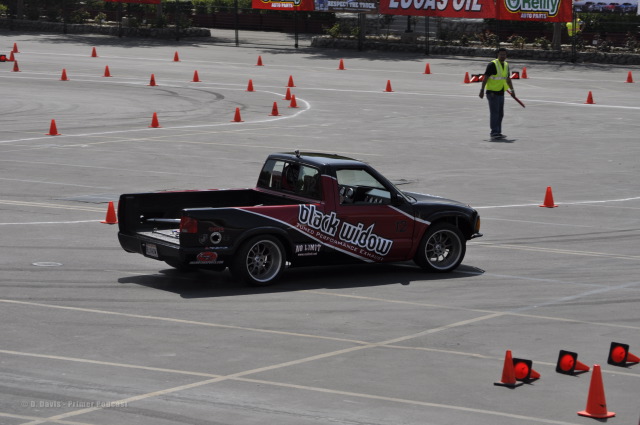The image depicts a black pickup truck labeled "Black Widow" in diagonal black letters with a white outline, positioned on what appears to be a practice track or parking lot. The road surface is gray, featuring straight white lines at the bottom and rounded white lines at the top, bordered by numerous orange cones. While two cones stand upright at the bottom right, three have fallen over. The truck's bed is missing, and it faces toward the right side of the image. A person wearing a yellow safety vest stands near the top right, holding a stick, possibly managing the cones. Additional details include a red, partially cut-off sign in the background and a fenced area, suggesting a contained setting. The overall scene is quite dim, giving a dark, gray tone to the surroundings.